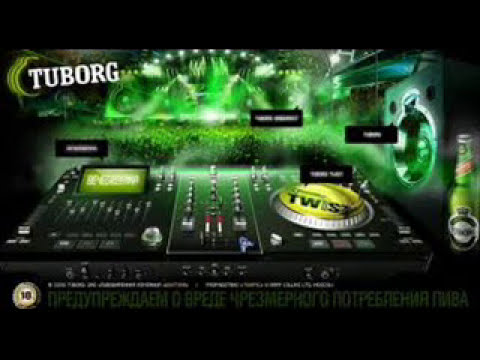This detailed illustration, possibly an advertisement for Tuborg beer, presents a dynamic snapshot of a concert from the perspective of a DJ or sound mixer. In the foreground, a sophisticated DJ setup with analog controls and a spinning lime-green record takes center stage. Surrounding this are various mixing board lights, enhancing the scene's vibrancy. On the right, a sleek green glass bottle of Tuborg beer with a twist-off cap and a black and silver label is prominently displayed. The background reveals a sea of enthusiastic concertgoers bathed in green lights emanating from the stage, emphasizing the lively atmosphere. The image, predominantly black and green to reflect the brand's colors, also features a caption in white reading "TUBORG" in the upper left corner. Large black and silver speakers bookend the scene, contributing to the high-energy, immersive concert vibe.